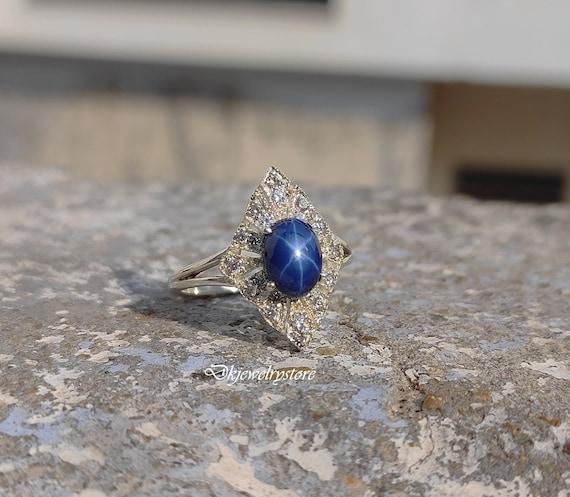This image captures a beautifully intricate silver ring placed on a distressed, multi-colored surface, possibly marble or concrete, adorned with specks of gray, white, and blue. The ring features a prominent diamond-shaped centerpiece, elegantly embedded with small diamonds. At the heart of this diamond shape, a large oval sapphire takes center stage, marked by thin white lines running vertically and diagonally across it, creating a striking X pattern. The ring's elegant design is accentuated by two prongs that hold the brilliant sapphire in place. A watermark with the text "DK Jewelry Store" appears beneath the ring in a flowing font. The background is slightly blurred, offering hints of other buildings or surfaces.